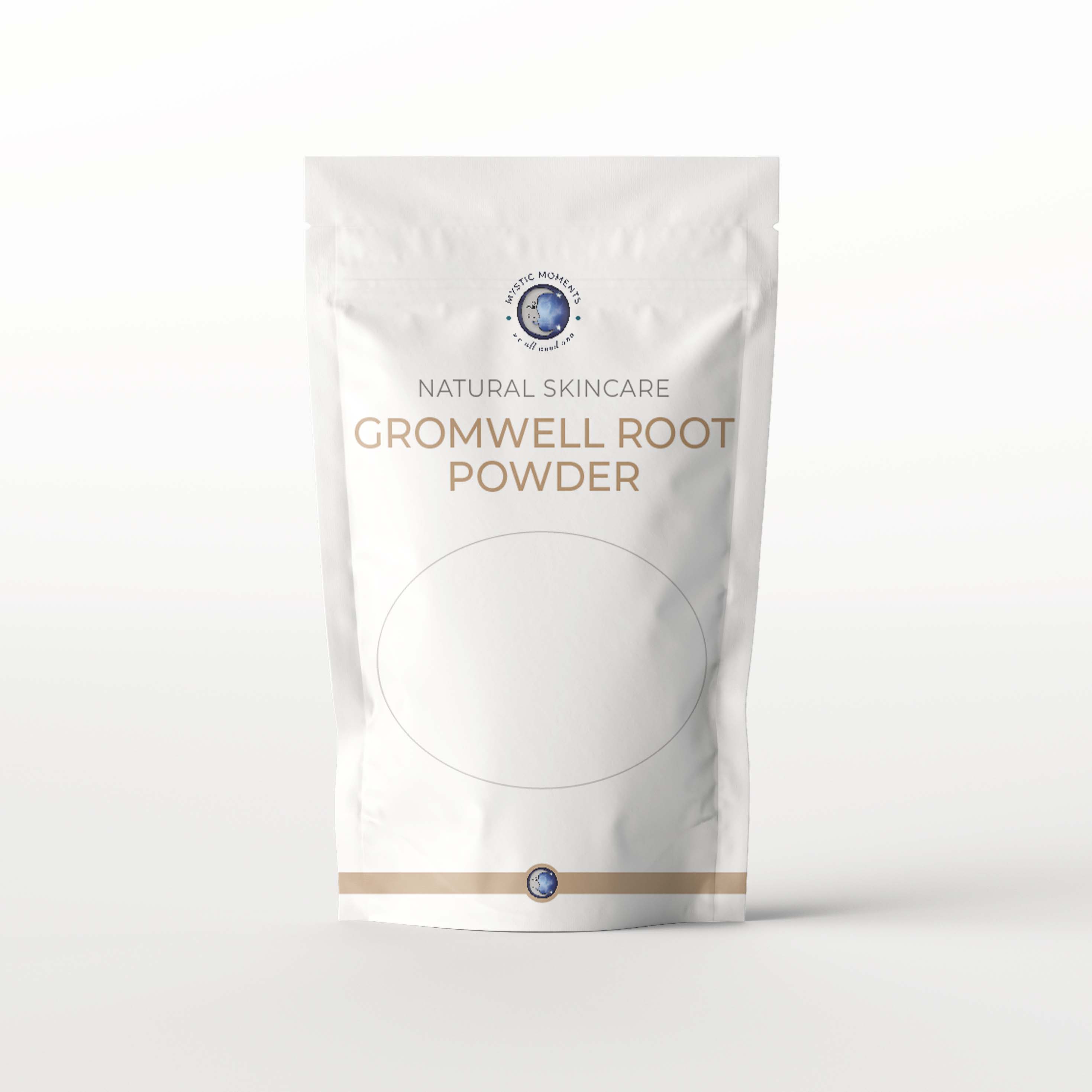The image is of a white, resealable package containing natural skin care product, specifically Gromwell Root Powder. The top portion of the packaging features a circular emblem with a half moon adorned with a human face, stars, and the earth beneath a night sky, alluding to a mystical theme. Above this emblem, the brand name "Mystic Moments" is displayed in black lettering. Below the emblem, in the middle section of the bag, “Natural Skin Care” is written in a gray-brown color, followed by “Gromwell Root Powder” in gold-brown lettering. The bag appears filled and is designed with a blend of soft gray fading into white in the background. The bottom section of the bag has a thin circle and repeats the moon and earth logo. The overall design suggests the product is likely marketed on a natural skin care site.